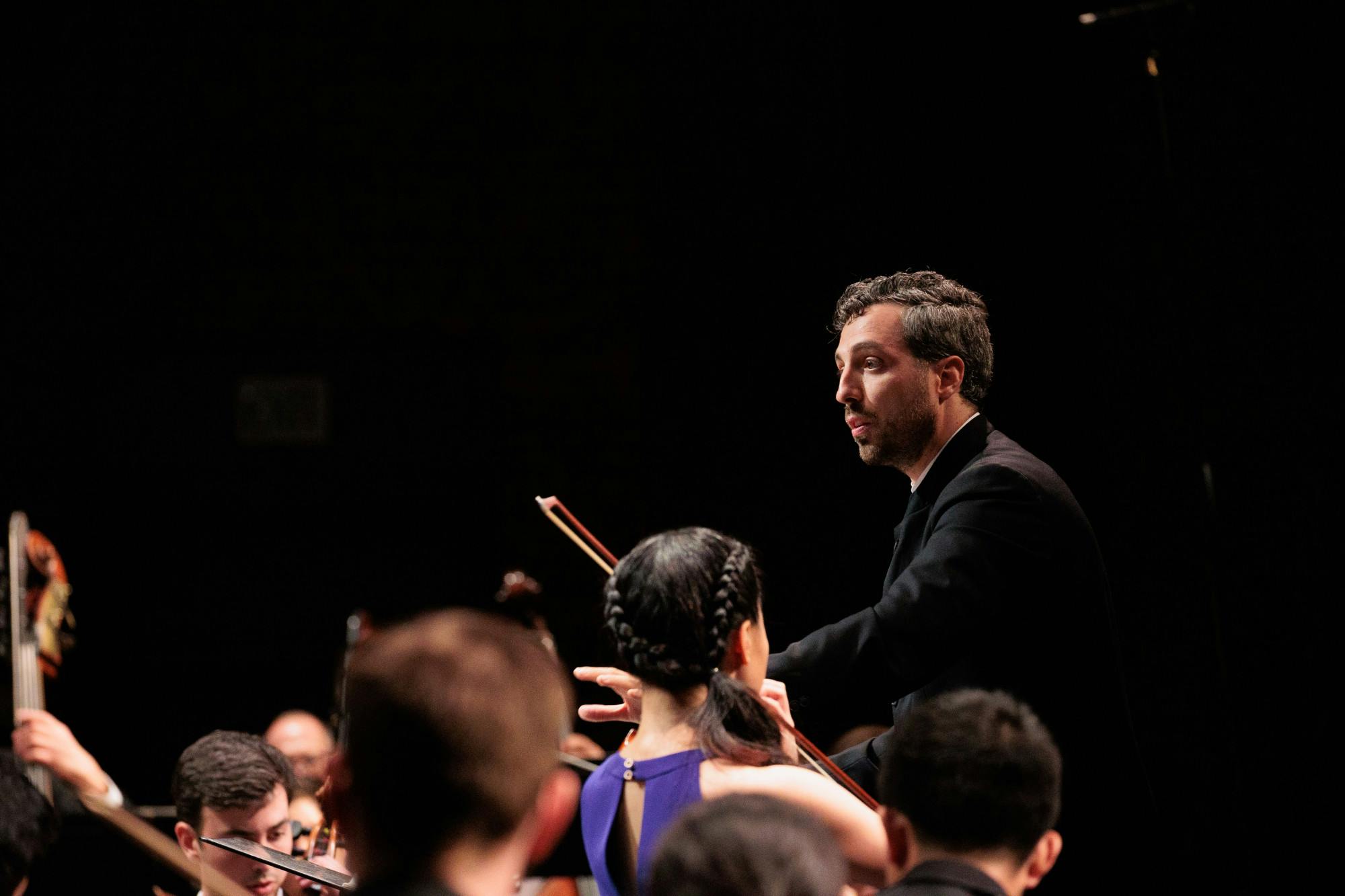This image captures a focused maestro conducting an orchestra against a pitch-black background. The maestro, a middle-aged man with salt-and-pepper hair and some stubble, is dressed in a black suit. He stands at the front, his hands outstretched as he directs the musicians before him. In the foreground, a young woman with braided brown hair, wearing a blue dress, stands as she plays a solo on her violin, suggesting she is the focus of the piece. You can see part of a cello on the left side and what appears to be a double bass in the background. The musicians, mostly seen from behind, are seated and deeply absorbed in their performance. The photograph, likely taken at a concert hall, is crisp and well-lit, highlighting the intensity and concentration of the orchestra during what seems to be a live performance or a rehearsal.